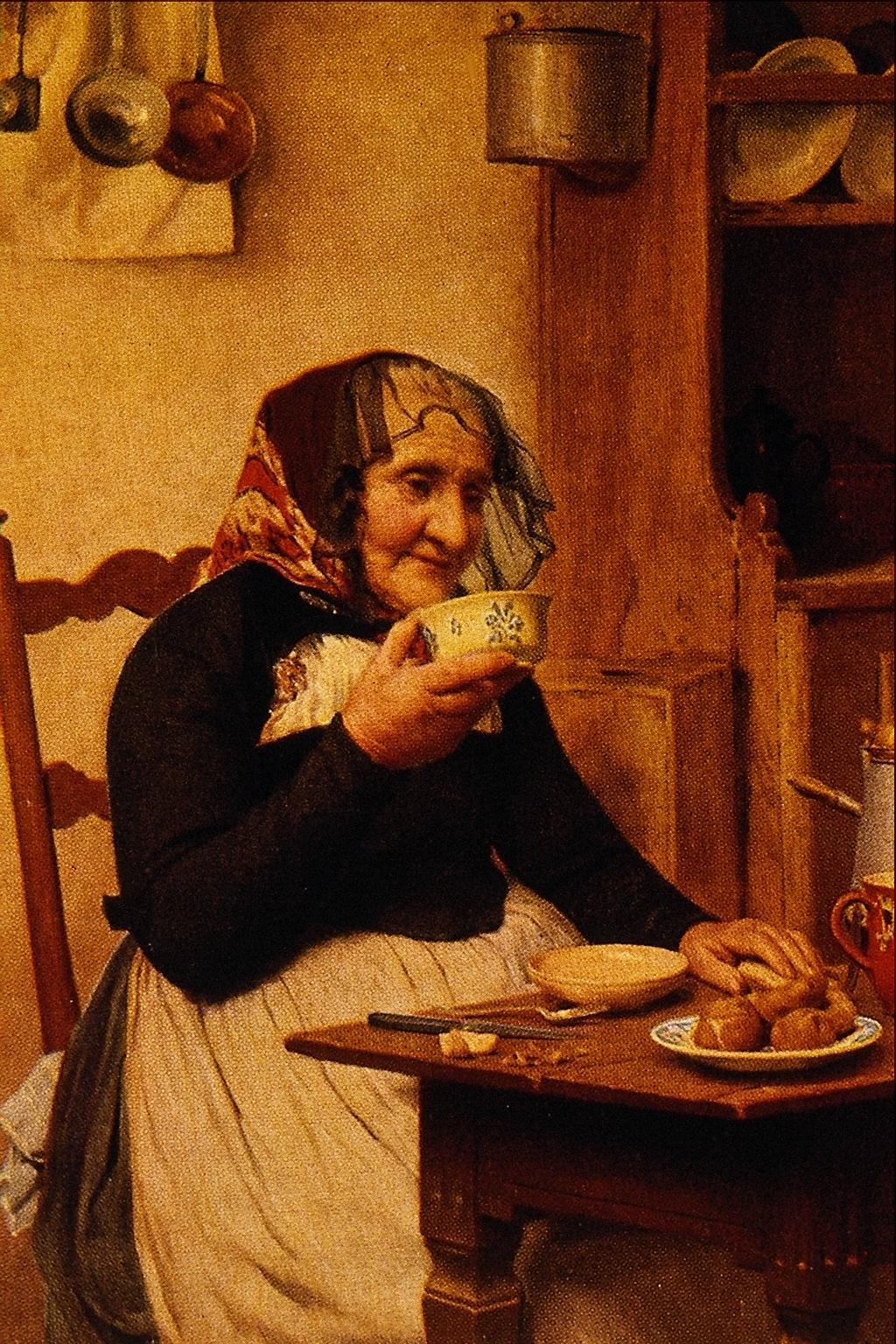This highly detailed and realistic painting portrays an older Caucasian woman seated at a brown wood farm-style table, exuding a lifelike quality akin to a photograph. Dressed in a black long-sleeve top, a black cap with a fringe around the brow, and a red print scarf behind it, she also wears a white apron tied around her waist. Her dark grey skirt is partially visible as she sits on a brown wooden ladder-back chair positioned on the left side of the image. The woman holds a cream-colored bowl, decorated with a design around the edges, close to her mouth, suggesting she is about to take a sip, possibly from a soup or some tea.

The scene captures a moment of contentment as she gazes downward with a smile, appearing happy and pleased. On the wooden table in front of her lies another cream-colored bowl, a plate with a few pieces of brown bread, and several utensils, including a spoon and a knife next to the plate. The setting indicates a meal, possibly lunch or breakfast, in a farmhouse kitchen. 

The background features a brown wood cupboard partially in view, holding two white plates and a silver kettle, along with ladles hanging on the wall above. The overall ambiance is one of rustic simplicity and domestic warmth, typical of farm-style portraiture realism.